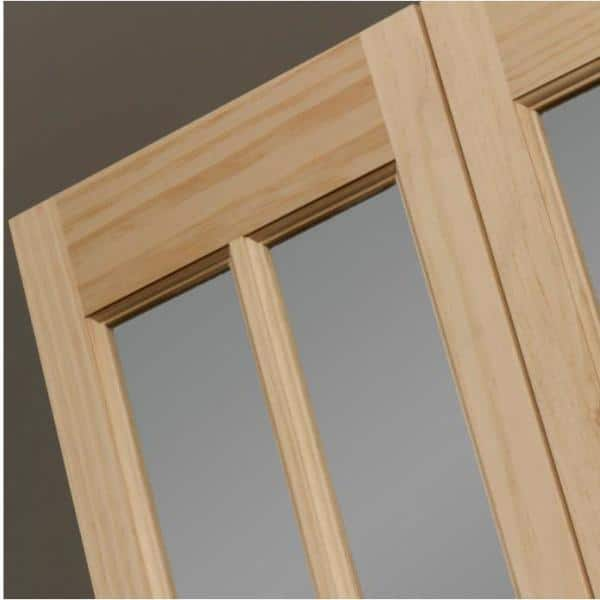The full-color photograph appears to be taken indoors, depicting a wooden door frame and partial view of a window system, possibly consisting of two doors or windows. The image is square with no discernible border or background, and the scene is captured at a slanted angle. The door frames and window panes are prominent, with the window glass having a non-transparent grayish tint. The wood around the frame is unvarnished, unstained, and unpainted, showcasing a natural grain pattern. There are two main windows visible, divided by a vertical board. The frame features a combination of tan, light brown, brown, and off-white tones. The ceiling and wall, both of a dark brownish color with smooth and flat textures, complete the background, subtly shifting the focus to the intricate details of the wood grain and the interplay of light and angles on the door frame and windows.